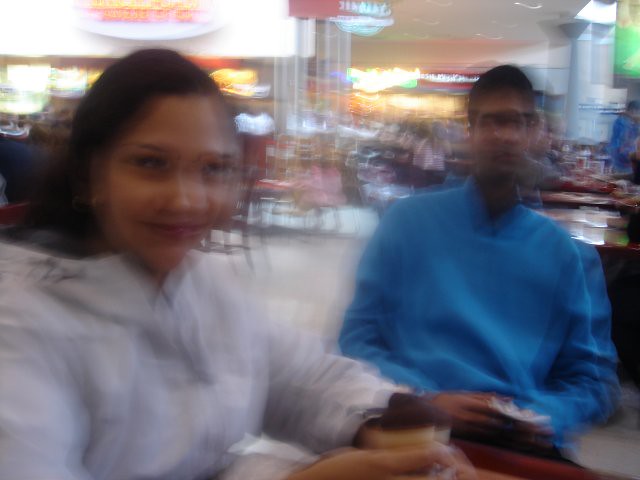An intensely blurred photograph captures two individuals seated in a vibrant food court. The blur is so prominent that it makes the image hard to view comfortably. On the left, a woman with brown hair and a radiant smile faces the camera. She wears red lipstick and a white hoodie and holds an ice cream cone filled with chocolate ice cream. The severe blur effect creates a doubled image of her face, with her nose appearing twice. Next to her sits a man in a blue long-sleeve shirt. His dark hair and head are distorted, blurring in multiple directions. The background is a hazy mix of white and red signs and indistinct people dressed in a variety of colors including white, red, pink, purple, and blue, all contributing to the overall blurred and dynamic scene.